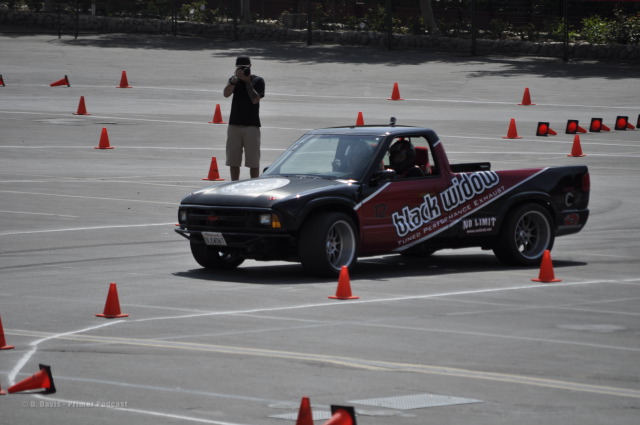In this detailed outdoor daytime photograph, a black pickup truck with a cab and an open bed dominates the center of a parking lot scattered with numerous traffic cones, some upright and some upended. The truck prominently features a red banner across its side, bearing the text "Black Widow" in bold black letters with a white outline. Below this, in smaller red text, it reads "Tuned Performance Exhaust" and "No Limit." The asphalt surface of the lot is marked with various white and gray lines and painted traffic indicators. 

A man, dressed in a black T-shirt and khaki shorts, stands next to the truck, appearing to hold a camera or phone, as he looks directly at the viewer. The background includes green trees that frame the upper part of the image, enhancing the sunny daytime setting. The overall color palette includes shades of black, gray, white, red, green, and orange, contributing to the vividness and clarity of this outdoor scene.